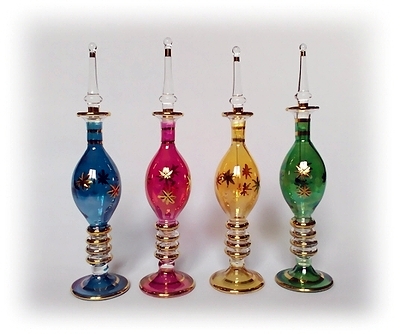The image features four intricately designed glass bottles, each displaying distinctive characteristics and arranged from left to right in the colors light blue, pink, yellow, and green. Each bottle exhibits an elegant, almost hourglass-like shape, enhanced with golden star patterns that graces their sides. They stand against a light gray background that softly transitions to white at the edges, creating a delicate contrast that highlights the bottles' vibrant hues.

Starting from the left, the light blue bottle has a circular base and a slender, elongating stem adorned with gold rings, which then widens into a bulb that is decorated with golden star motifs. Next is the pink bottle, similarly structured with a pink base that flows into a gold-ringed stem and a star-patterned bulb. The yellow bottle follows, mirroring the blue bottle in design with its own complement of gold rings and star decorations. Finally, the green bottle stands on the far right, sharing the same elegant form and decorative elements as its companions.

Crowning each bottle is a tall, slender glass cap, adding a touch of sophistication to their design. The overall presentation is captured against a smooth, almost ethereal gray background that adds depth, with subtle reflections and shadows of the bottles projected upon it, emphasizing the bottles' striking appearance.